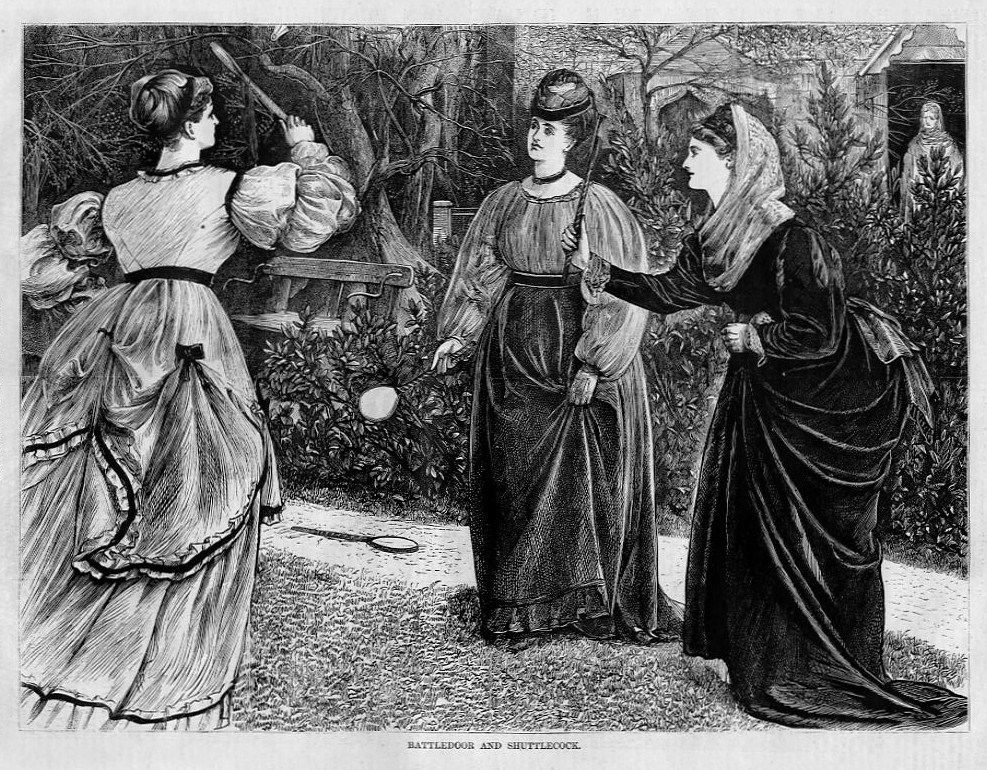This black and white drawing, titled "Battle Door and Shuttlecock," captures a detailed Victorian-era scene with three women engaged in a game using tiny paddles, reminiscent of flyswatters. They are elegantly dressed in full-length gowns, with one woman on the left having her hair tied up, the center woman wearing a small hat and a choker, and another on the right with her head wrapped in a loose cloth. The women are positioned in a park-like setting with bare trees, bushes, and a wooden bench in the background. One paddle lies on the ground beside them. In the far right background, a woman is seen standing in a doorway, possibly watching the game. A statue stands at the edge of the scene, contributing to the old-fashioned ambiance of the setting.